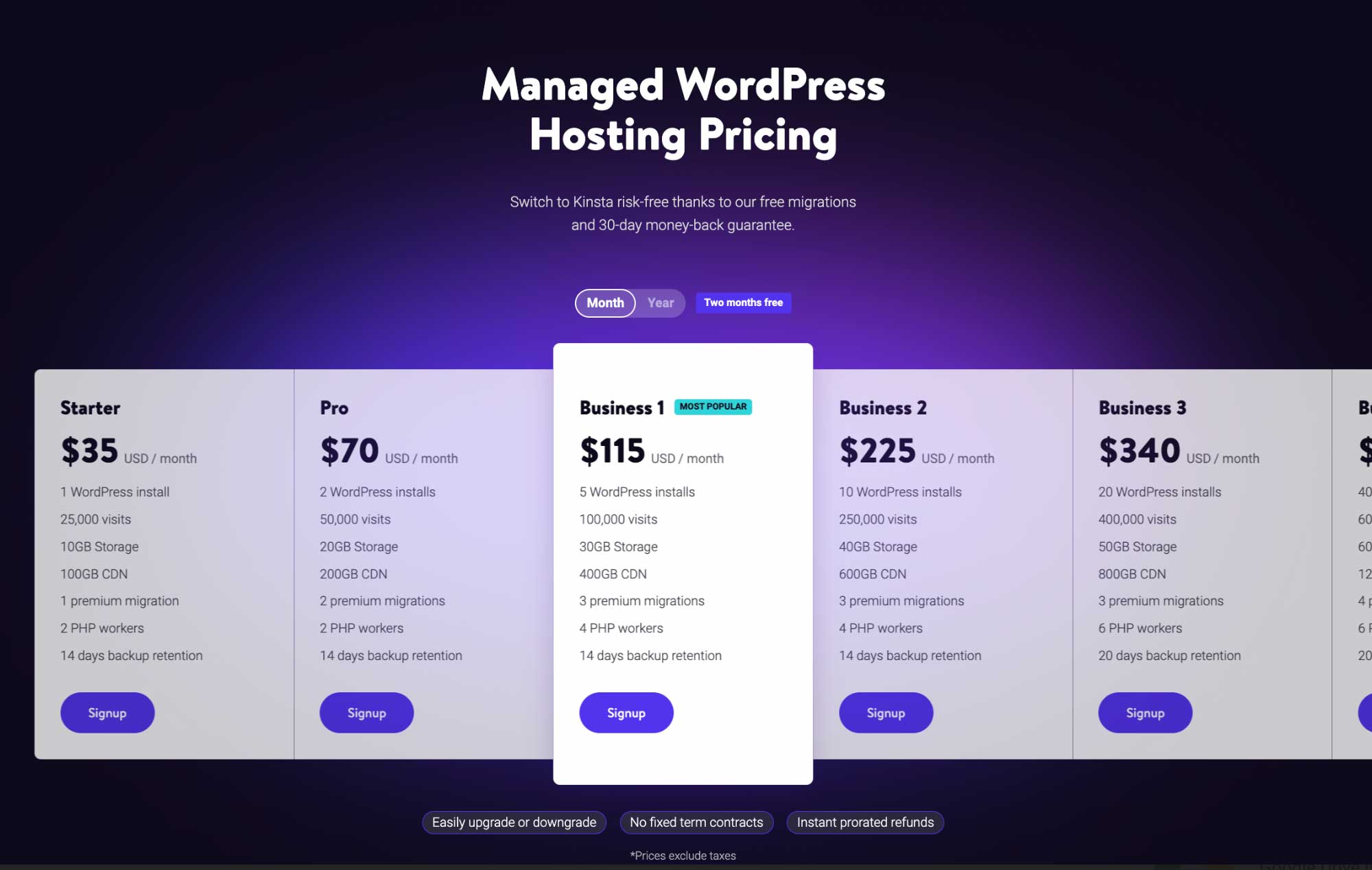The image is a screenshot of a computer screen displaying the pricing plans for Kinsta's managed WordPress hosting. The screen has a deep bluish-purple background, which accentuates the clarity of the white text in the center. The central message reads: "Switch to Kinsta risk-free thanks to our free migrations and 30-day money-back guarantee." 

Directly below this message, users have the option to select either monthly or yearly payment plans, with a note indicating that opting for the annual plan grants two months free. 

On the far left of the pricing table, the "Starter" plan is listed, priced at $35 per month. This plan includes a detailed list of its features underneath. Moving to the right, the "Pro" plan is displayed at $70 per month, also accompanied by a comprehensive feature list. 

In the center, the "Business 1" plan is highlighted as the "most popular," priced at $115 per month. Next to it are the "Business 2" and "Business 3" plans, priced at $225 and $340 per month, respectively. At the bottom of each pricing column, there is a bluish-purple "Sign Up" button for easy navigation.